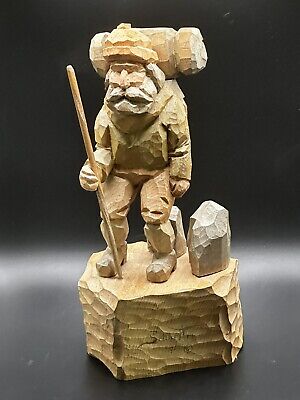The image depicts a detailed wood carving of a mountain man, likely carved from a light beige or light tan wood. The sculpture shows the man in mid-step, walking with a hiking stick held in his left hand. He sports a prominent mustache and a beard, and he wears a hat. On his back, there is a backpack with a notably larger sleeping bag secured on top. The carving is mounted on a slightly cylindrical base, which contains some writing starting with the letter "S" that is not fully legible. Surrounding the man are several gray rocks near his feet. The statue is positioned on a dark gray surface, set against a pitch-black background with white coloring visible above, suggesting a light source.